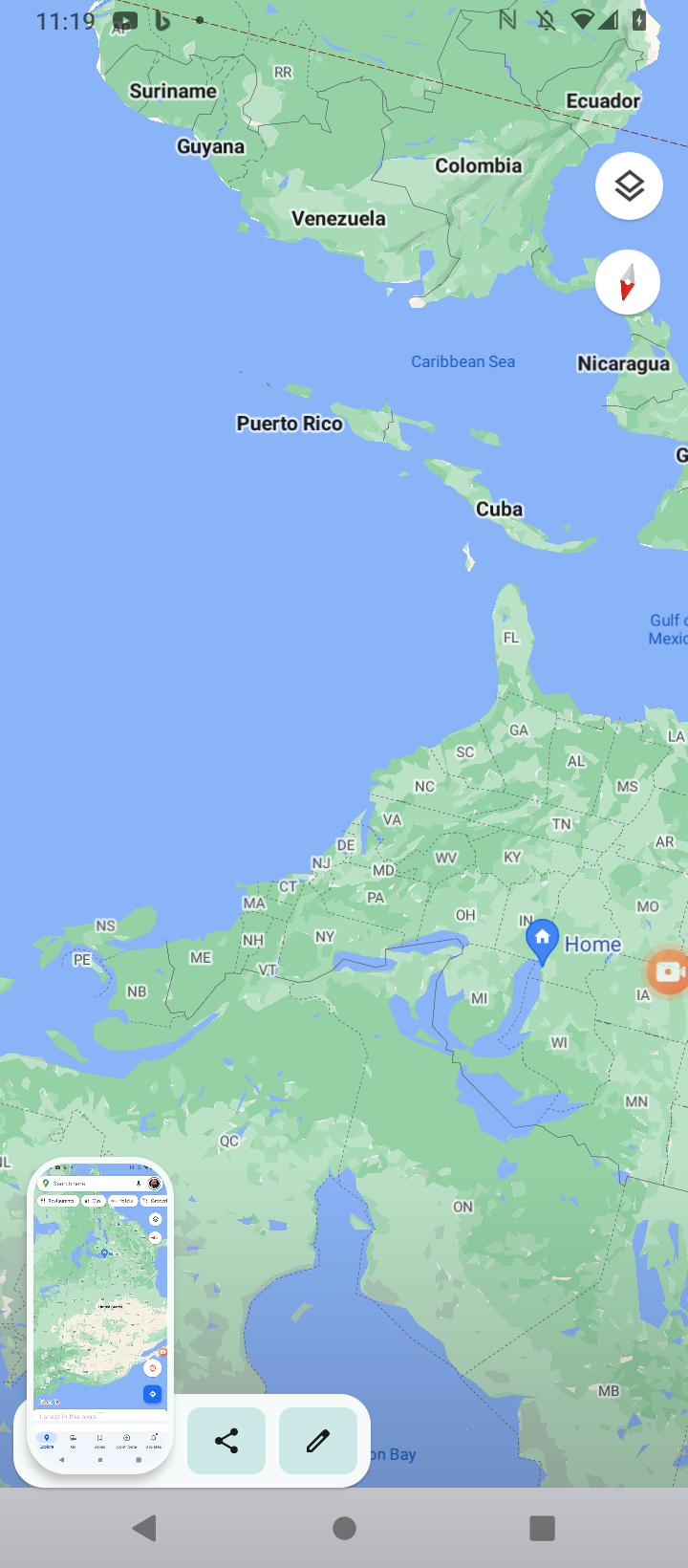This image is a detailed screenshot from an Android phone, showcasing a map from possibly Google Maps. The navigation bar at the bottom is gray with three darker gray buttons: a left-pointing back arrow, a circular home button, and a square for recent apps – indicative of an older Android interface. The transparent notification bar at the top features a clock displaying 11:19, Wi-Fi and battery indicators, an alarm signal, and a YouTube notification, with notifications turned off.

The map itself is an unusual depiction of North and South America, with South oriented towards the top and North towards the bottom, making familiar geographies appear inverted: Canada is at the bottom, Florida at the top, and Cuba and Puerto Rico in the middle. The map displays locations like Suriname, Guyana, Venezuela, Colombia, and Ecuador prominently, along with U.S. states such as New York, Ohio, Indiana, and Wisconsin, indicating a broad geographical focus.

A notable feature of the screenshot is an image of another phone overlaying the bottom left-hand corner, giving the appearance of a phone within a phone, which includes a user's profile image in its top right corner. Additionally, there is a white oval at the top left with icons for sharing and editing the image. The map also highlights the user's home location near Indiana.